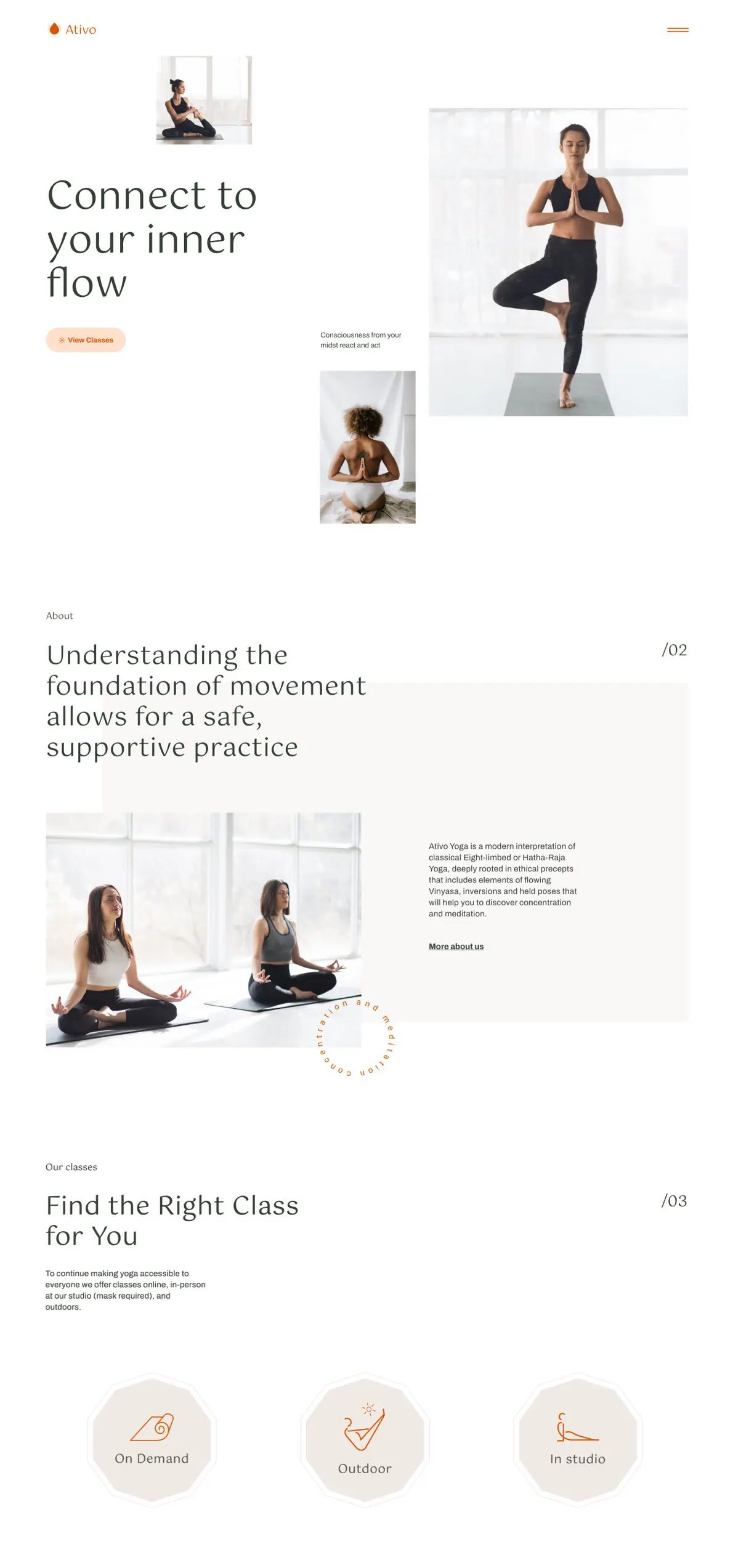The image features a clean, white background with various elements associated with yoga and a brand named "ATIVO." In the upper left-hand corner, there is an orange shape resembling a water drop or teardrop, beside which the text "ATIVO" is written in uppercase letters. On the opposite side, two orange horizontal lines stretch across the top.

Below this, on the left-hand side, there's a photograph of a woman performing a yoga pose. She is dressed in black yoga pants and a black top, with her hair tied up in a bun. She is positioned on what appears to be a gray yoga mat, with one leg bent and the sole of her foot turned inward. 

Beneath this image, the text "CONNECT TO YOUR INNER FLOW" is written in black, with "CONNECT TO" in uppercase. An orange oval shape is visible, within which "View Classes" is printed in a darker orange hue.

Further down, there is an intriguing image of a woman seen from the back, who appears to be topless, though no details of her front are visible. She is wearing white underwear and holding her hands together in a prayer position behind her back. Above this image, another woman, identical to the first, is seen standing on one foot, dressed in the same black yoga attire with her hands clasped together and eyes closed.

To the left of these images, a detailed description explains the philosophy of Ativa Yoga: "Understanding the foundation of movement allows for safe, supportive practice. Ativo Yoga is a modern interpretation of classical eight-limb or Hatha Vajra Yoga deeply rooted in ethical precepts that includes elements of flow and vinyasa, inversions and forces that help you discover concentration and meditation." The section concludes with a text prompt, "More about us."